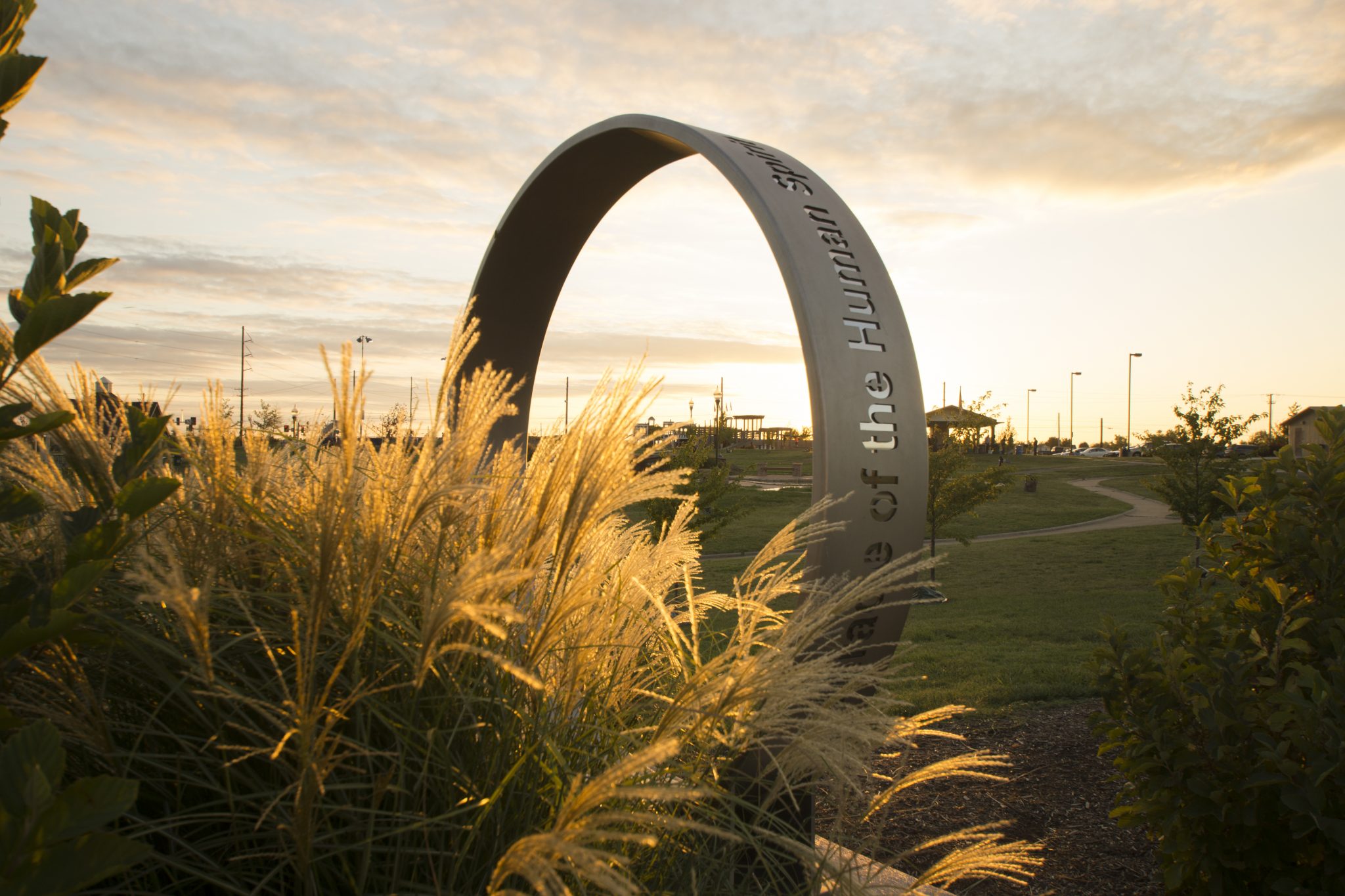In this horizontally-oriented photograph taken at sunset, the scene is imbued with warm hues of gold, yellow, and dusky pink. The foreground features a dark, dirty mulch area, where various plants are growing. Taking center stage is a large, gray, three-dimensional sculpture representing the human spirit. This ring-like sculpture has engravings on the outer edge, and although it's unclear if it forms a complete circle or ends on a flat surface, it arches gracefully much like a rainbow.

Beyond the sculpture, the park landscape opens up with lush green grass and several pavilions. In the middle of the ring’s open space, a wooden playground structure is visible in the distance, inviting children to climb and play. To the right, lights illuminate a parking lot crowded with cars. The overall composition captures a serene yet lively park scene, brought to life under the enchanting colors of the setting sun.